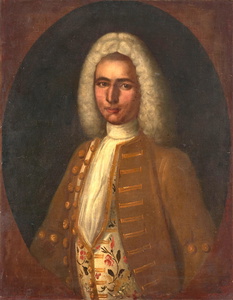The image features a detailed frontal portrait of an older Caucasian gentleman, likely from the 17th century, wearing a white wig and dressed in period attire. He dons a dark tan overcoat adorned with multiple circular buttons along the left side and the elbow areas. The right side of his overcoat is characterized by stripes. Beneath the overcoat, he wears a floral vest with intricate patterns in gold, red, brown, and black, and a white undershirt, which may actually be a white ascot or scarf that thickens at the bottom with brown edges matching the jacket. The portrait is framed within a black oval set against a brownish square background, suggesting the gentleman had posed for this painting that exudes an intense, perhaps judicial or court-like character. His lips appear to have some deformities, adding a unique aspect to his dignified demeanor.